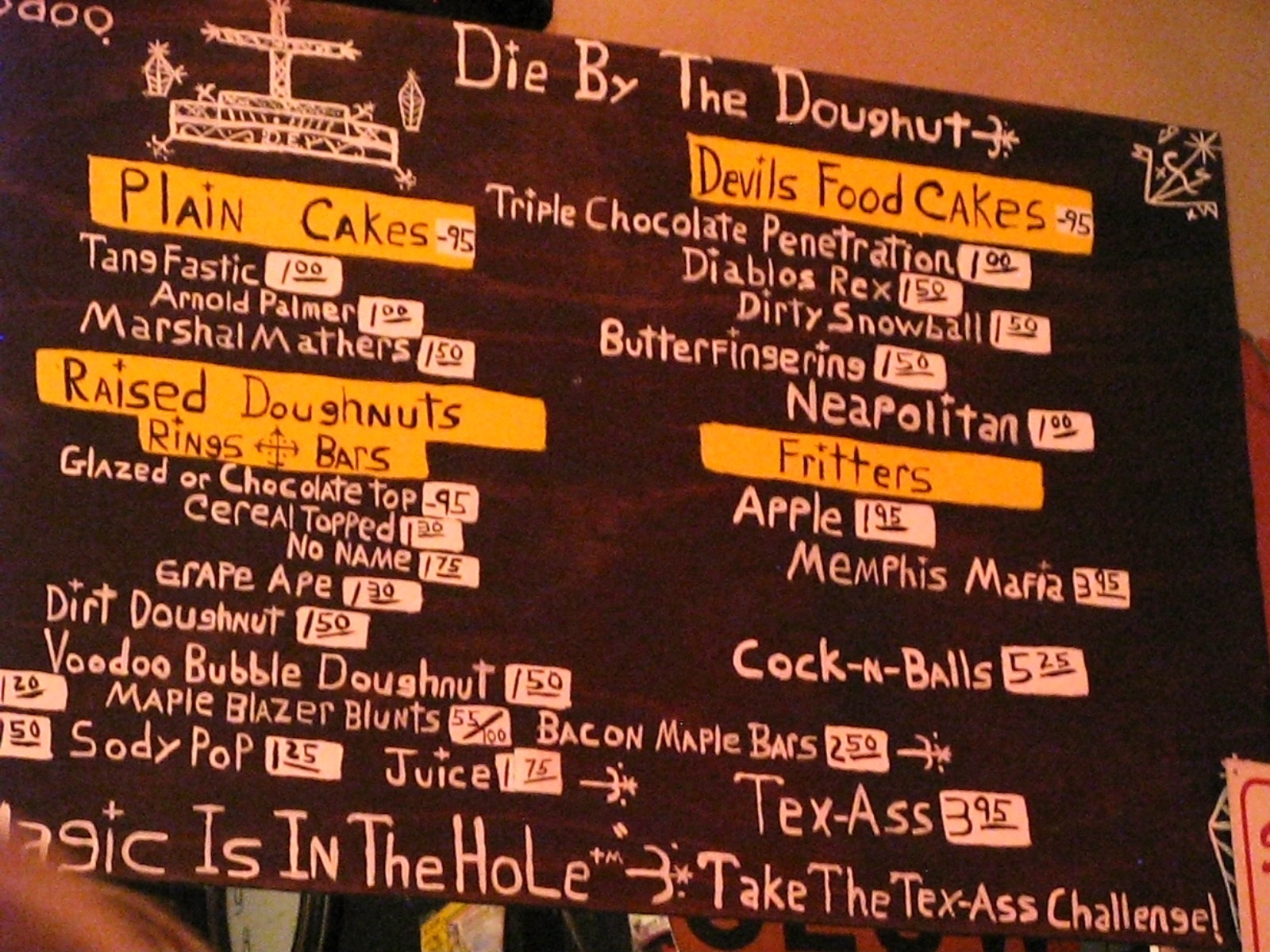The image depicts a menu displayed on a board affixed to a wall, likely within a bakery or bakeshop. The menu title, "Dye by the Doug Nut," is elegantly written in intricate, stylized handwriting that mixes uppercase and lowercase letters, implying a certain creative flair.

The menu is divided into several distinct sections, each highlighting different types of baked goods:

1. **Plain Cakes**: This section lists various plain cake options.
2. **Raised Donuts**: Here, the menu offers raised donuts in the form of rings or bars, with options such as Glazed or Chocolate.
3. **Devil's Food Cakes**: This section presents rich, chocolate devil's food cake variations.
4. **Fritters**: Various types of fritters are also available.

Unique and enticing names populate the menu, including:

- **Tangfastic**
- **Arnold Palmer**
- **Plain Cakes**
- **Raised Donuts**
- **Glazed or Chocolate Devil's Food Cakes**
- **Dirty Snowball**

Additional quirky and specialty items include:

- **Voodoo Bubble Donut**
- **Maple Blazer Blunts**
- **Sody Pop** (S-O-D-Y Pop)
- **Juice**
- **Tex-Ass**

At the bottom of the menu, a playful sign reads, "Magic is in the Hole," followed by an intriguing challenge: "Take the Tex-Ass Challenge." This challenge appears to be related to a specific menu item named "Tex-Ass."

The overall presentation of the menu, with its variety of options and whimsical names, suggests a fun and unique bakery experience.